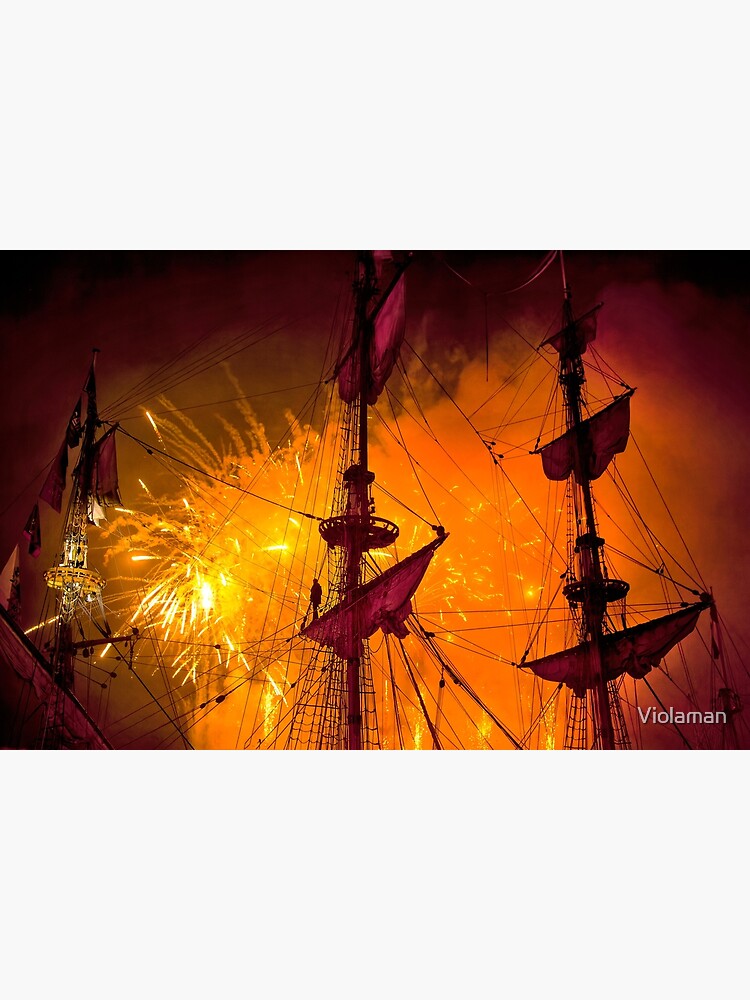The image captures a photorealistic, close-up view of three dark red sails of a ship, possibly a pirate or historical vessel, set against a dramatic backdrop of fiery explosions or fireworks in the sky. The vibrant, bright orange sky is filled with smoke and light, contrasting sharply with the dark black areas surrounding the fireworks. The sails are only partially unfurled and are crisscrossed with many ropes and wires. Just beneath one of the crow's nests, a solitary figure is visible standing above a sail. In the lower right corner, the text "Viola Man" is present, likely indicating the artist or photographer. The composition is dominated by hues of maroon, orange, and gold, with light sparks from the fireworks creating a vivid focal point towards the left side of the image. The scene is richly detailed, suggesting a night filled with pyrotechnic spectacle against a historical maritime setting.